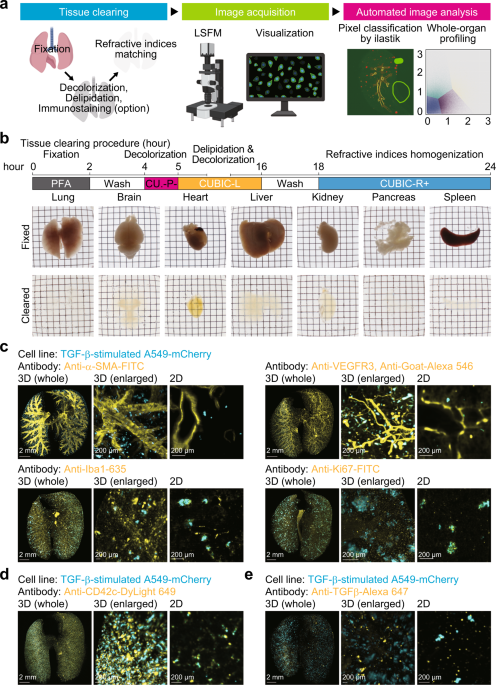The image is an informational chart detailing a medical imaging and analysis procedure. At the very top, it features a heading labeled "A." Below it, a blue rectangle with white text reads "Shoot Clearing," followed by a green rectangle with white text indicating "Image Acquisition." Subsequently, a pink rectangle with white text states "Automated Image Analysis."

Beneath these text labels, there is a picture of cartoon lungs illustrating steps like "Fixation," "Decolorization," "Delipidation," "Immunostaining Option," and "Refractive Indices Matching." Adjacent to this, a microscope image labeled "LSFM" is shown. Below the microscope, there is an image of a computer monitor captioned "Visualization," which is connected to the description "Pixel Classification by Elastic Whole Organ Profiling."

The subsequent section labeled "B" details a "Tissue Clearing Procedure" and includes steps such as "Hour Fixation," "Decolorization," etc. The chart incorporates multiple colors to differentiate its elements, such as shades of blue, green, lime green, pink, light orange, yellow, gray, black, and white. Sections C, D, and E are positioned underneath sections A and B, forming a comprehensive medical diagram for tissue analysis and imaging processes.